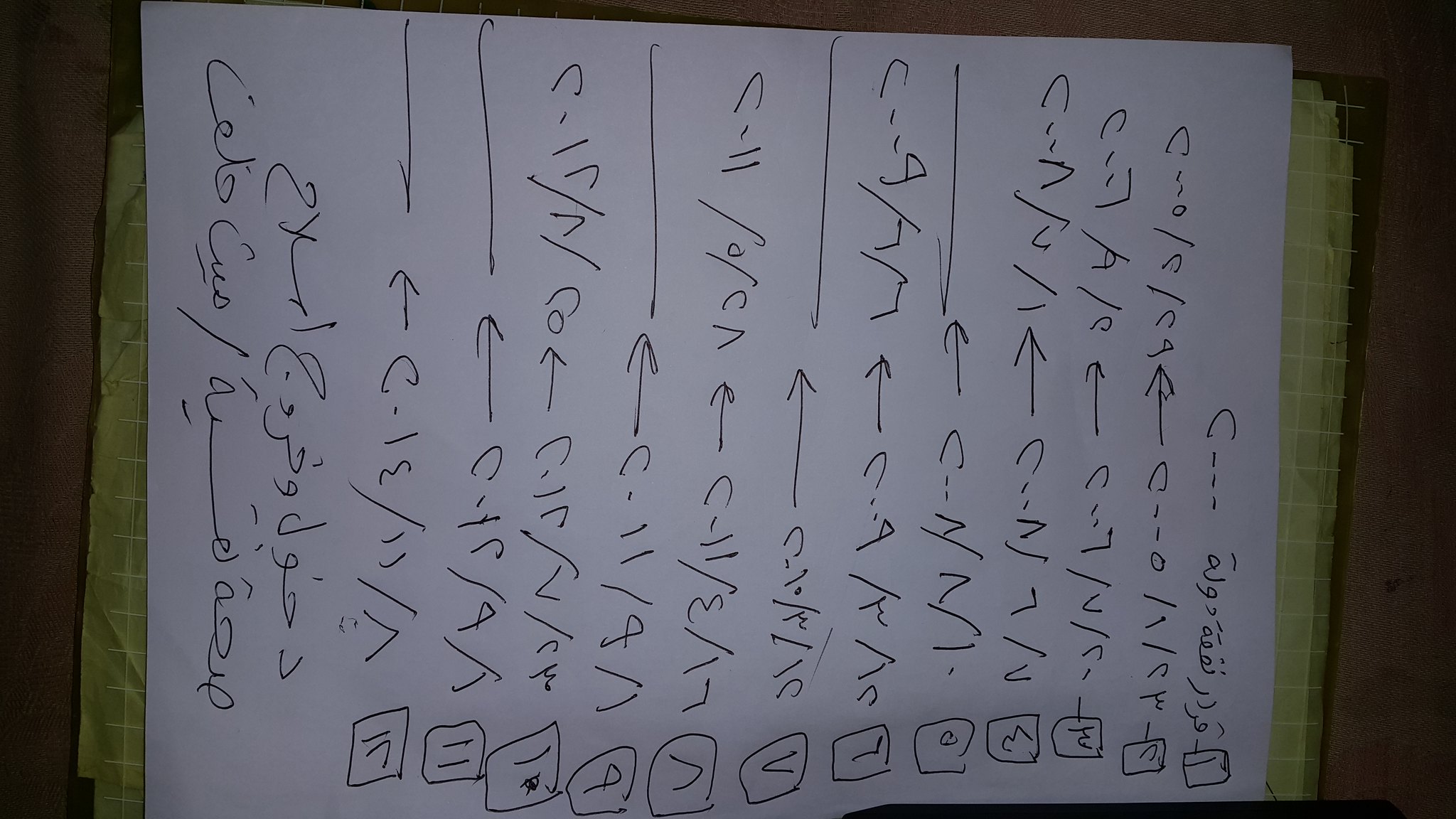This photograph features a piece of white paper resting atop a green and white striped towel, which could either be a kitchen or bathroom towel. The towel itself is placed on a tan surface, possibly a kitchen cabinet, though the specific piece of furniture is indeterminate from the image. The white sheet of paper is covered with an array of letters and shapes arranged in a vertical line. An arrow directs attention to these elements, followed by some text and various small square boxes that seem like they are intended for answers or responses. Among these boxes, some contain numbers such as '9' and '11', while others feature mathematical symbols like greater than or less than signs. Interestingly, there appears to be a shape that resembles a backward Z. The orientation of the paper adds a layer of ambiguity, as there are elements on both sides, making it challenging to determine the correct side for viewing. No textual indication helps clarify the intended orientation of the paper.